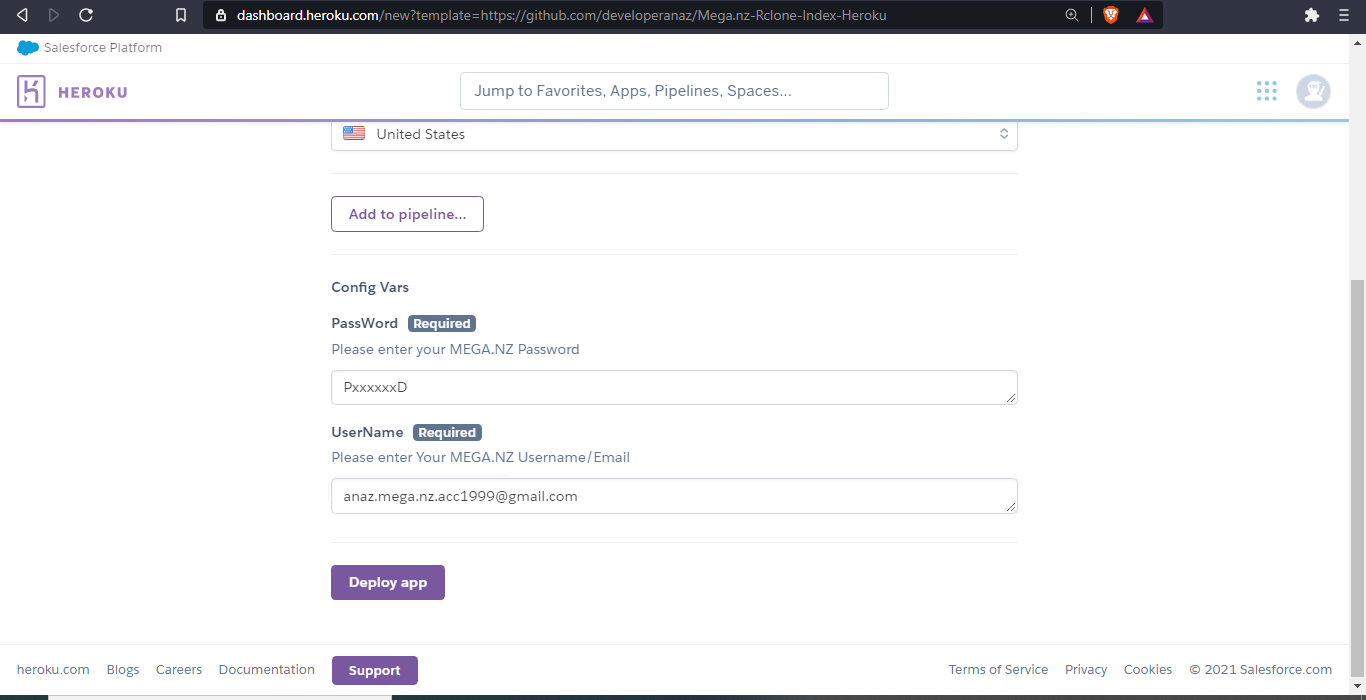The image depicts a screenshot of a Heroku website dashboard. The header features a black bar with the URL "dashboard.heroku.com." In the top left corner is the Heroku logo, which consists of a purple image resembling two L's placed together with two lines within a box. Directly underneath, there is a search bar labeled "Jump to" accompanied by options including "Favorites," "Apps," "Pipeline," and "Spaces."

On the right-hand side, the header contains two light, faded icons and a dropdown menu defaulted to "United States," which is adjustable. Below this, a purple button labeled "Add to pipeline" is prominently displayed. Adjacent to it, the text "Config Vars, password required" in black informs users to enter their "Mega NZ" password and username. 

Additionally, a purple box labeled "Deploy app" in white text is situated below these fields. At the bottom of the page, a purple "Support" button with white text is present. The footer on the left-hand side includes links to "Heroku.com," "Blogs," "Careers," and "Documentation," while the right side lists "Terms of Service," "Privacy," "Cookies," and notes that the content is © 2021 Salesforce.com.